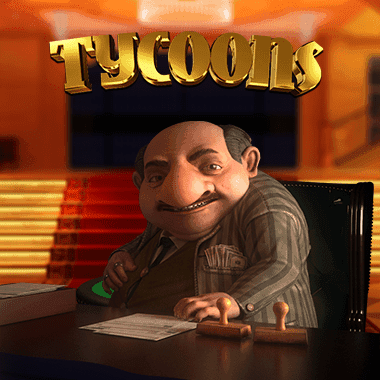This vivid image showcases a computer-generated, three-dimensional cartoon man at the center, distinctly characterized by his cartoonishly large nose and pronounced mustache. His appearance is notably disheveled with a bald top and tufts of brown hair above his ears, complemented by prominent sideburns. The man exudes a sly, almost leering expression, with a smile that hints at mischief. His brown eyes peek out from above his broad nose, enhancing the peculiar charm of his round, squat physique. Dressed in a vertically striped suit, which alternates between dark gray and brown tones, he embodies an aura of wealth and authority, emphasized by numerous dollar bills spilling out of his breast pocket and rings adorning his right hand. He sits before a desk scattered with papers, a book, and two wooden stamps, and a box to his side. He is seated in an ornate black chair, with a striking backdrop of red-carpeted steps leading up to a blurred black square. The background overall is a mix of warm hues, including tan, peach, brown, orange, and gold. Above him, in bold, shiny gold lettering, the word "Tycoons" asserts his likely affluent status, hinting at the conceptual theme of the image.